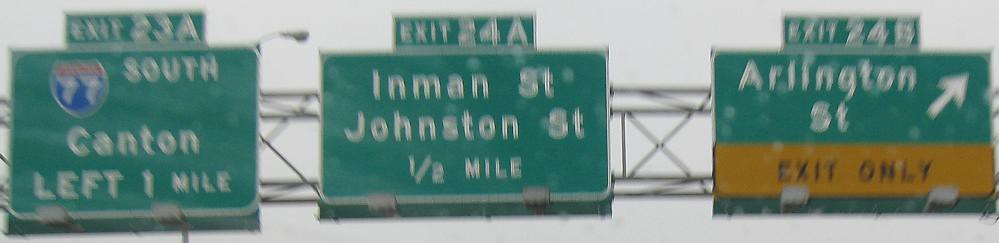The image depicts a series of highway signs along a major interstate, likely with multiple lanes of traffic. The first sign reads "Exit 23A, Interstate 77 South, Hampton, left 1 mile." The second sign indicates "Exit 24A, Inman Street and Johnston Street, half a mile." The final sign is for "Exit 24B, Arlington Street," featuring an arrow pointing to the right and labeled "Exit Only," suggesting that drivers should stay in the correct lane to exit. The signs are displayed against green backgrounds, typical for highway signage. The sky above is gray, indicating overcast conditions, but the ambient light suggests it is daytime. The overall scene hints at a bustling interstate, though no vehicles are visible in the captured frame.